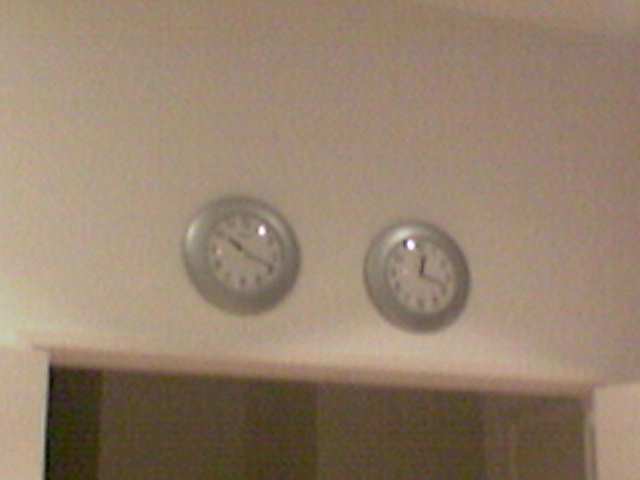This slightly blurry image captures two clocks mounted on a white wall above a doorway. The precise width of the doorway is indeterminate, leaving it unclear whether it leads to a larger space like a conference room or is a standard residential doorway. To the right, part of an adjacent door is visible. Both clocks feature identical silver or gray casings. The first clock, on the left, shows the time as 10:20, while the second clock, on the right, displays the time as 12:20. This suggests that one clock indicates a different time zone, potentially serving the needs of room occupants who operate in multiple time zones.